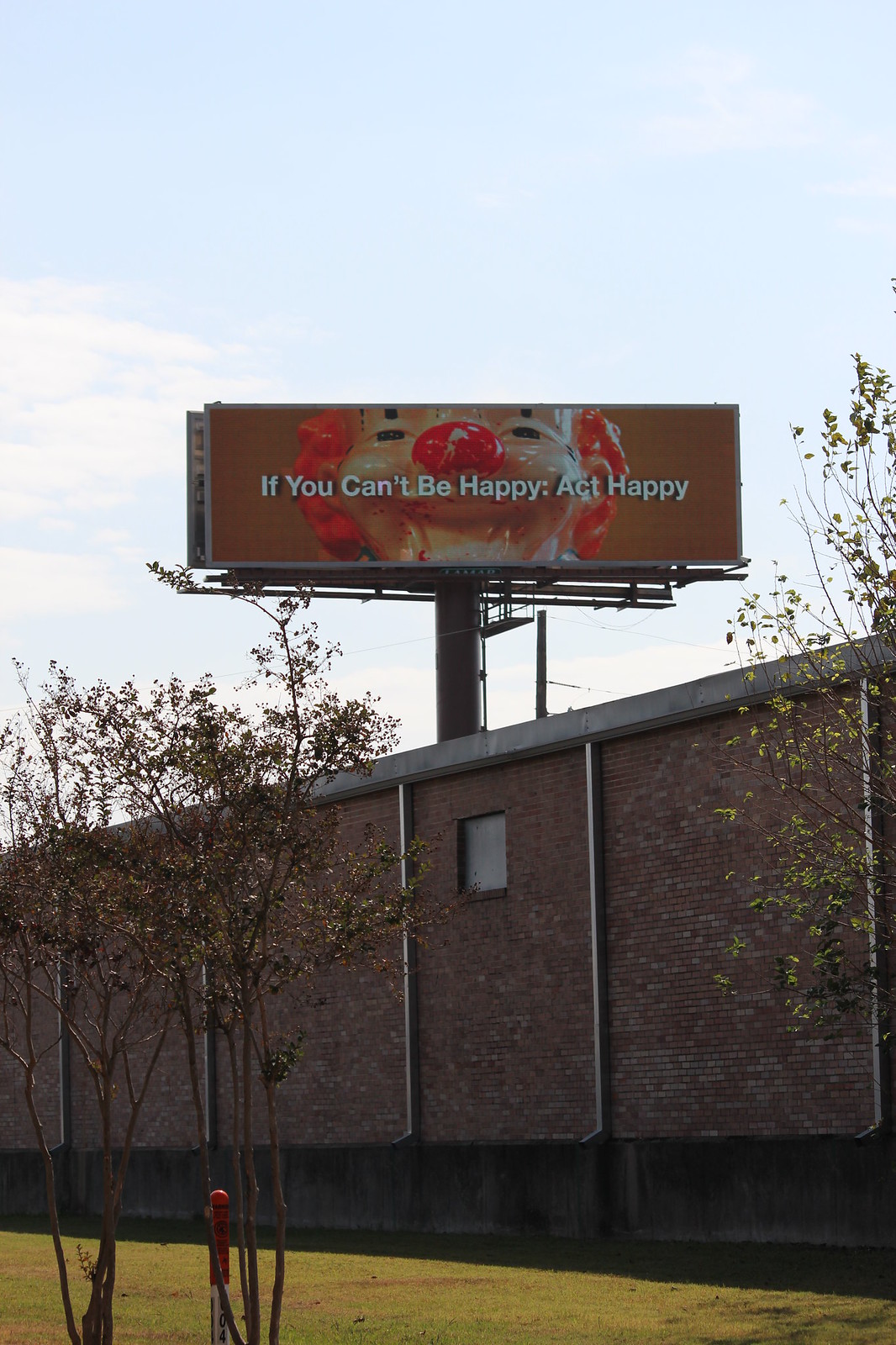In this shadowy daytime photograph, the viewer’s perspective is directed toward a distant billboard that stands tall beyond a brick building. The foreground is adorned with a patch of bright, sunlit grass, where two sapling-sized trees and a few scrawny branches on the right side cast delicate shadows. The brick building, located directly ahead, has a deep shadow enveloping its base. Approximately three-quarters up the height of the wall, a small, square window punctuates the uniformity of the bricks. Beyond the building, the billboard is mounted on a large, cylindrical pillar. The rectangular billboard features a brown background with the illustration of a large clown face accompanied by the caption, "If you can't be happy, act happy." The scene is set against a backdrop of a pale blue sky speckled with soft clouds.